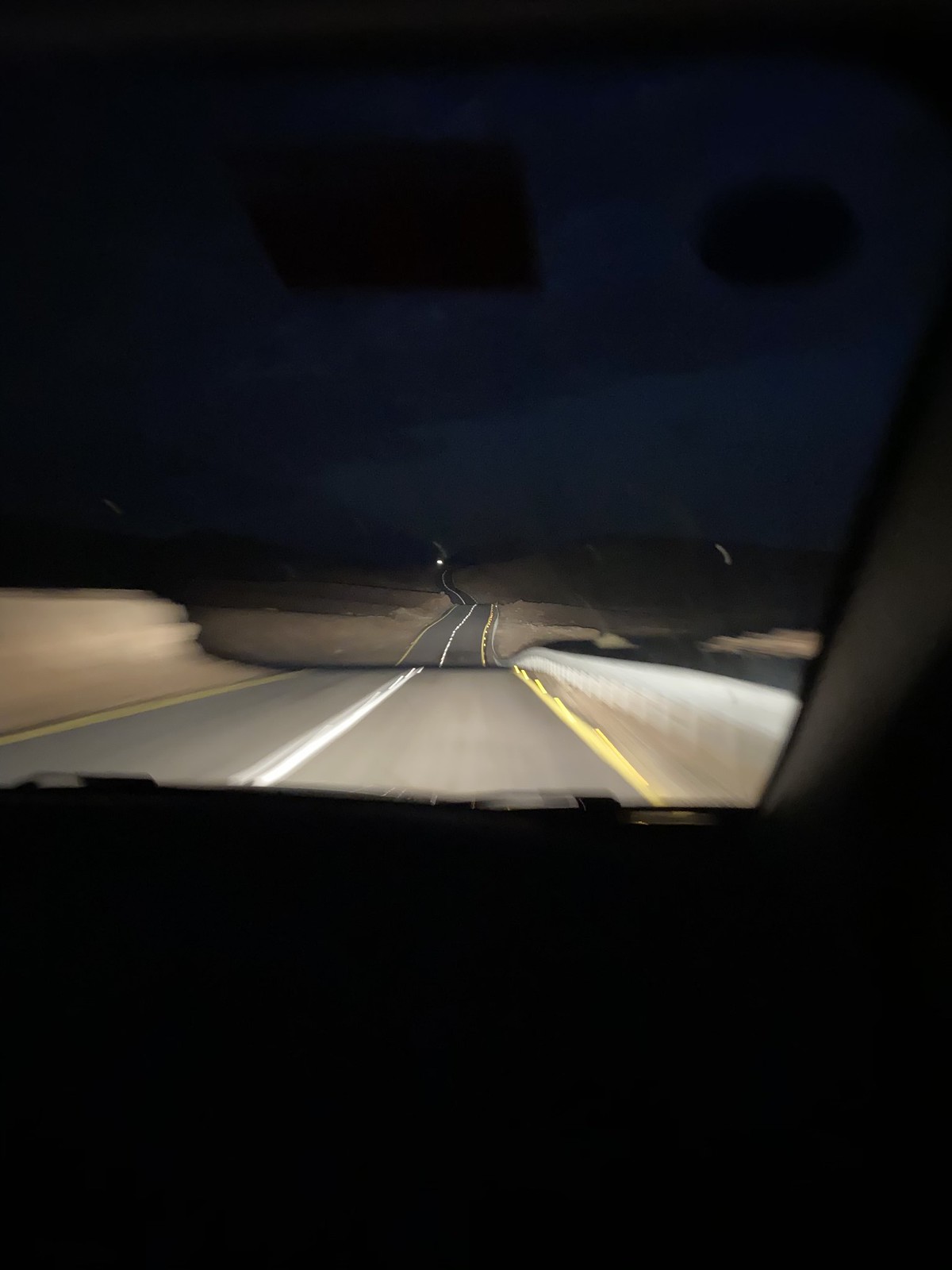This nighttime photograph captures a roadway from the perspective of the right front seat inside a moving vehicle. Visible are the car’s interior elements such as the windshield pillar and a dark silhouette of a windshield wiper near the camera. The view extends down a medium gray asphalt road, illuminated by the vehicle's headlights, and stretches into the horizon where a very dark blue sky with faint clouds reflecting light can be seen. The scene suggests a winding road that travels into the distance. The road features a solid white line down the center and a yellow solid line to the right, bordered by a steel guardrail on the right side. The land surrounding the roadway is predominantly bare dirt, resembling a desert landscape at night.